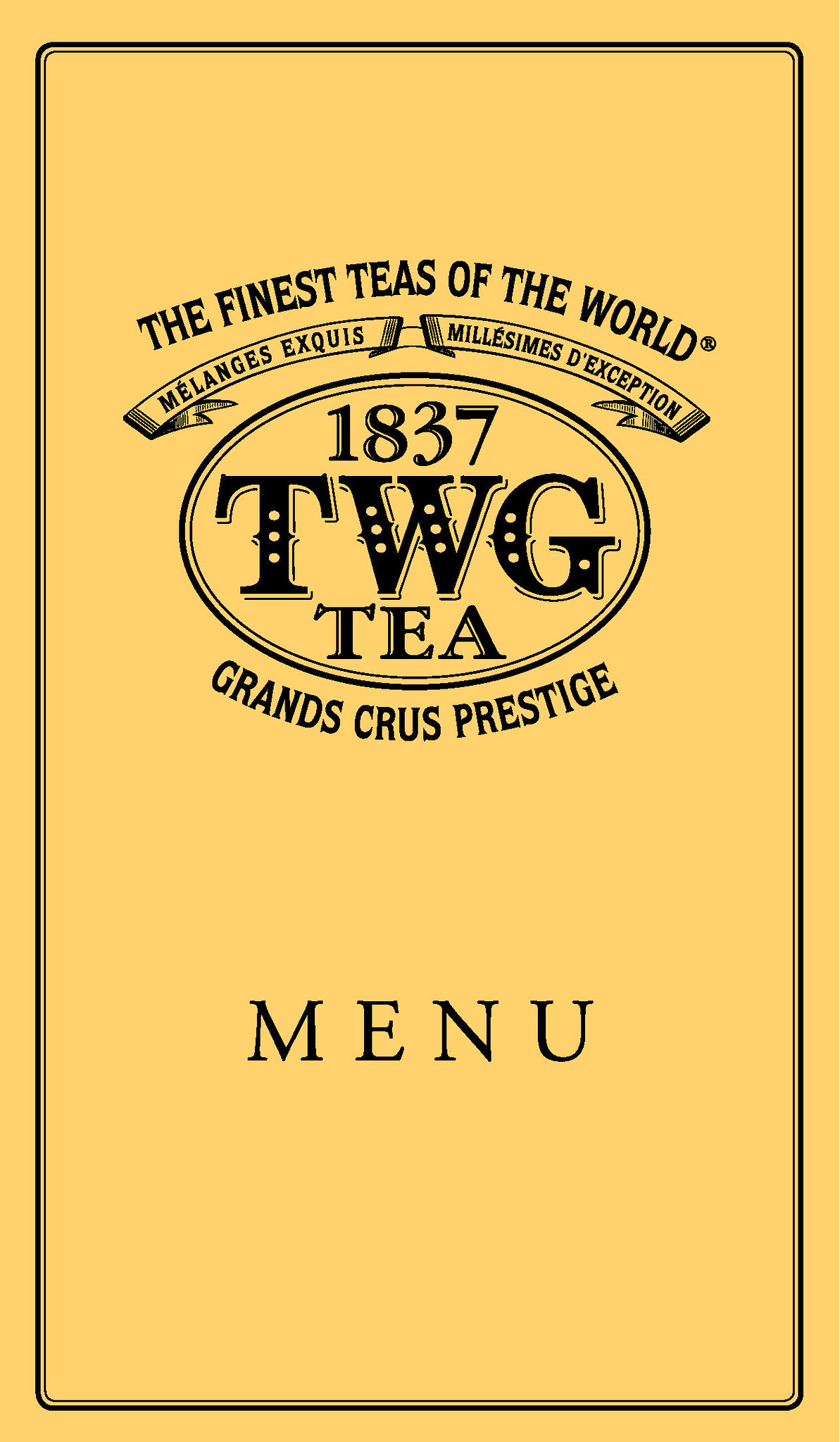This image displays the cover of a menu prominently featuring "The Finest Teas of the World." The menu is predominantly yellow with a fine black border, double-lined pinstripes surrounding the edge. At the top, the text reads "The Finest Teas of the World." Below this, a printed banner includes Spanish phrases "Melanges Isquiz" and "Mailissus de Excepcion." Centrally placed is an oval emblem with "1837 TWG T" inscribed, followed by "Grand Cruise Prestige." At the bottom, in bold black letters, the word "MENU" is displayed. All the text is in black, contrasting starkly against the yellow background. The borders culminate in rounded points at each corner, enhancing the formal aesthetic of the menu cover.